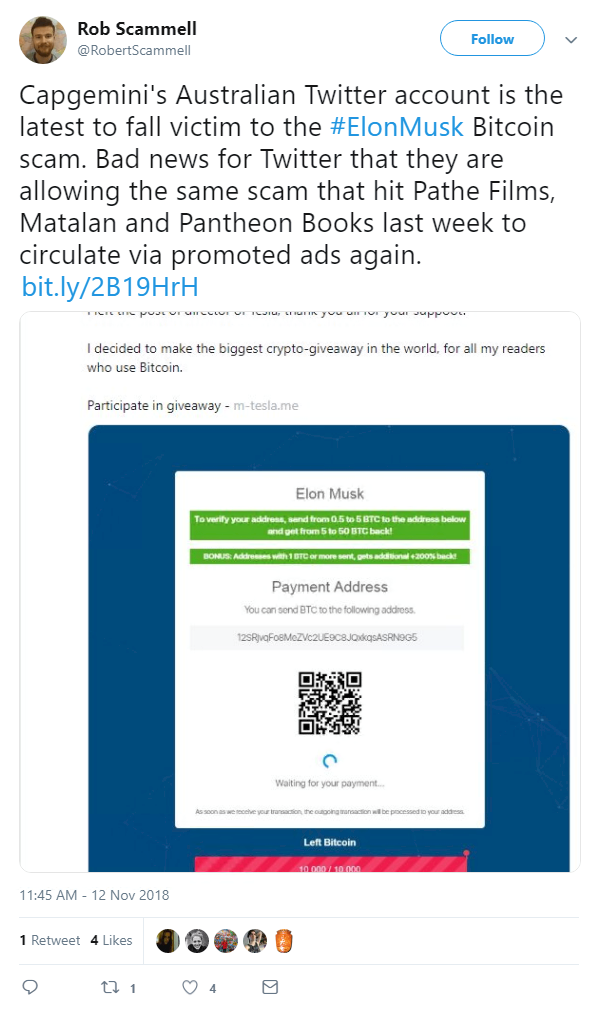The image appears to be a screenshot from a computer screen, predominantly featuring content on a white background. At the top, there is a circular profile picture of a man with dark hair and a beard. To the right of the picture, the name "Rob Scammell" is displayed in black text, and below it, in light gray, is the handle "@RobertScammell". To the right of this is a blue elliptical button with the word "follow" written in blue text inside it.

Below this section, there is some descriptive text. The first line reads, "Capgemini's Australian Twitter account is the". The subsequent text reads, "latest to fall victim to the #ElonMuskBitcoin scam." Notably, "#ElonMusk" and "Bitcoin" are highlighted in blue, while the rest of the text is in black. The text continues to describe the scam, stating, "Bad news for Twitter that they are allowing the same scam that hit Pathé Films, Matalan and Pantheon Books last week to circulate via promoted ads again." This is followed by a blue hyperlink, "bit.ly/2B19HrH".

Further down, there are two lines of darker text. Below this text, there is a navy blue, slightly rectangular section. Within this navy blue area, there is a white square that begins with the name "Elon Musk" in gray. Below this is a thick lime green bar with white text, followed by a slightly thinner lime green bar, also with white text.

Underneath the navy blue section, on the white background again, it states, "Payment address" in gray text, followed by two more lines of gray text. The image also features a QR code, partially overlaid with a blue half-circle and additional text below it. At the very bottom of the navy blue rectangle, there appears to be the top portion of another section that is colored red.